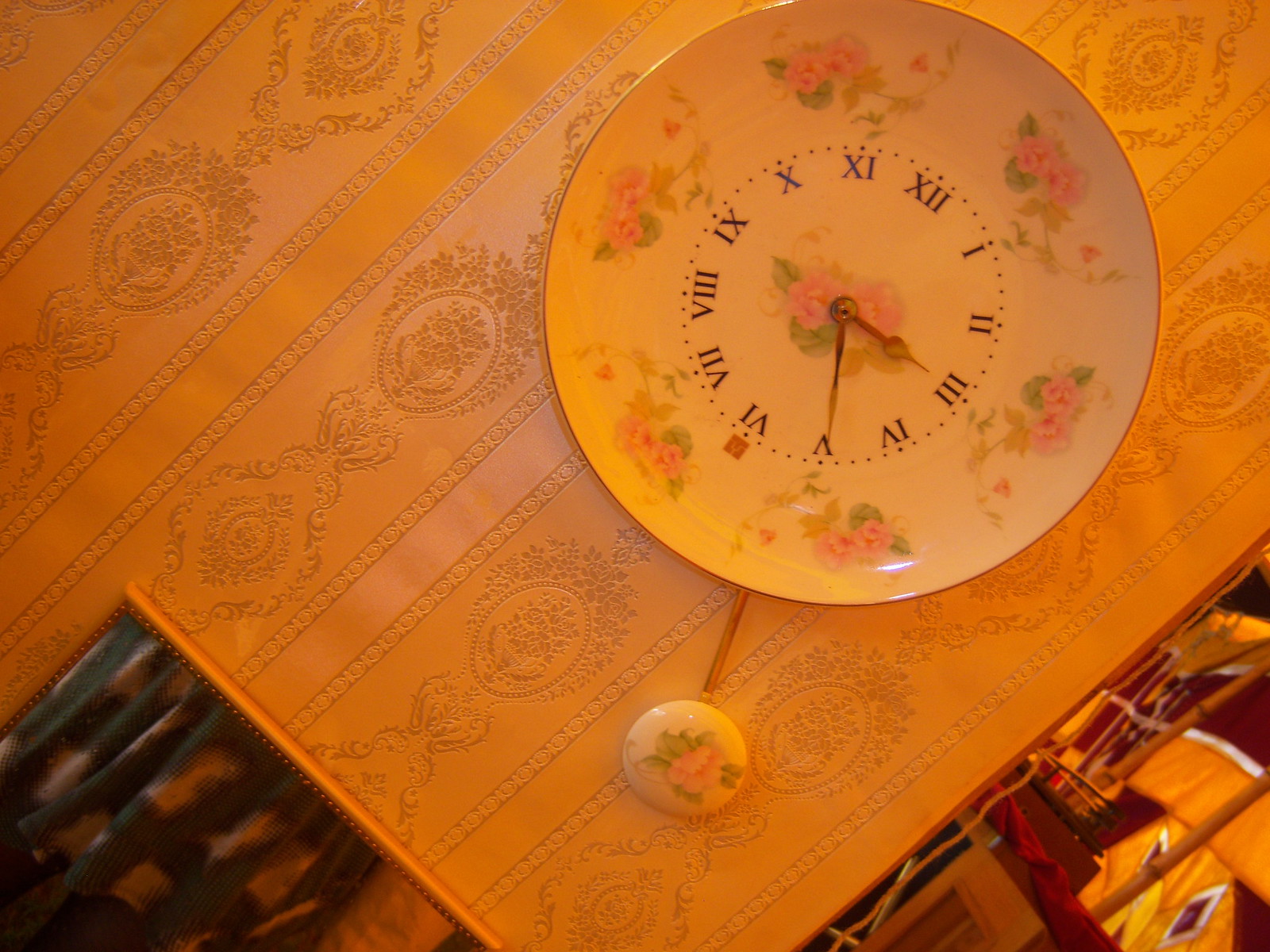This image shows an ornate, vintage-style clock fashioned from a fine china dinner plate, adorned with delicate pink rosebuds along the edges. The central face of the clock features Roman numerals from I to XII, and the current time displayed is 3:25. The minute and hour hands appear to be crafted from light-colored metal. Suspended below the clock is a gold wire holding a pendulum, also made from matching china with a single rosebud design. The clock hangs on a wall covered in luxurious, golden-yellow wallpaper with vertical stripes and intricate design elements resembling hand mirrors. However, due to the slightly tilted angle of the photograph, the wallpaper stripes run diagonally from the bottom left to the upper right. There are some indistinct objects in the bottom left and right corners of the image, with the one on the right appearing to be yellowish-orange banners.